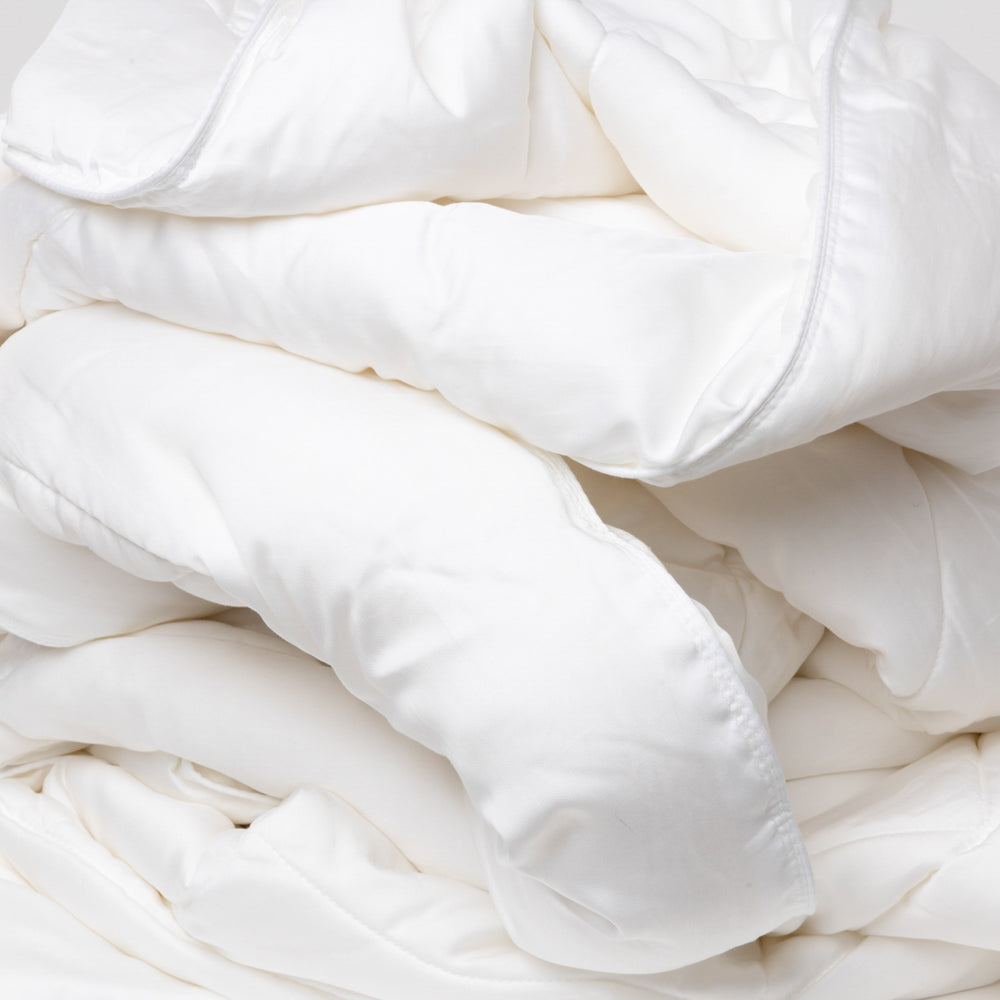The image depicts a large, white comforter, likely a billowy duvet, intricately folded and draped in a sinuous pattern. Illuminated by a warm white light from the front left, the soft and inviting fabric is accentuated, creating a contrast with the slightly shadowed right side. The stitching is clearly visible, adding a touch of detail to the plush, spotless surface. The comforter appears exceptionally fluffy, suggesting an inner filling of feathers or a similarly soft material. Multiple layers give an impression of being multiple comforters stacked together, with a portion of the top layer curling over, revealing the sumptuous inside. The overall scene is dominated by this voluminous, freshly laundered duvet, creating a cozy and inviting atmosphere.